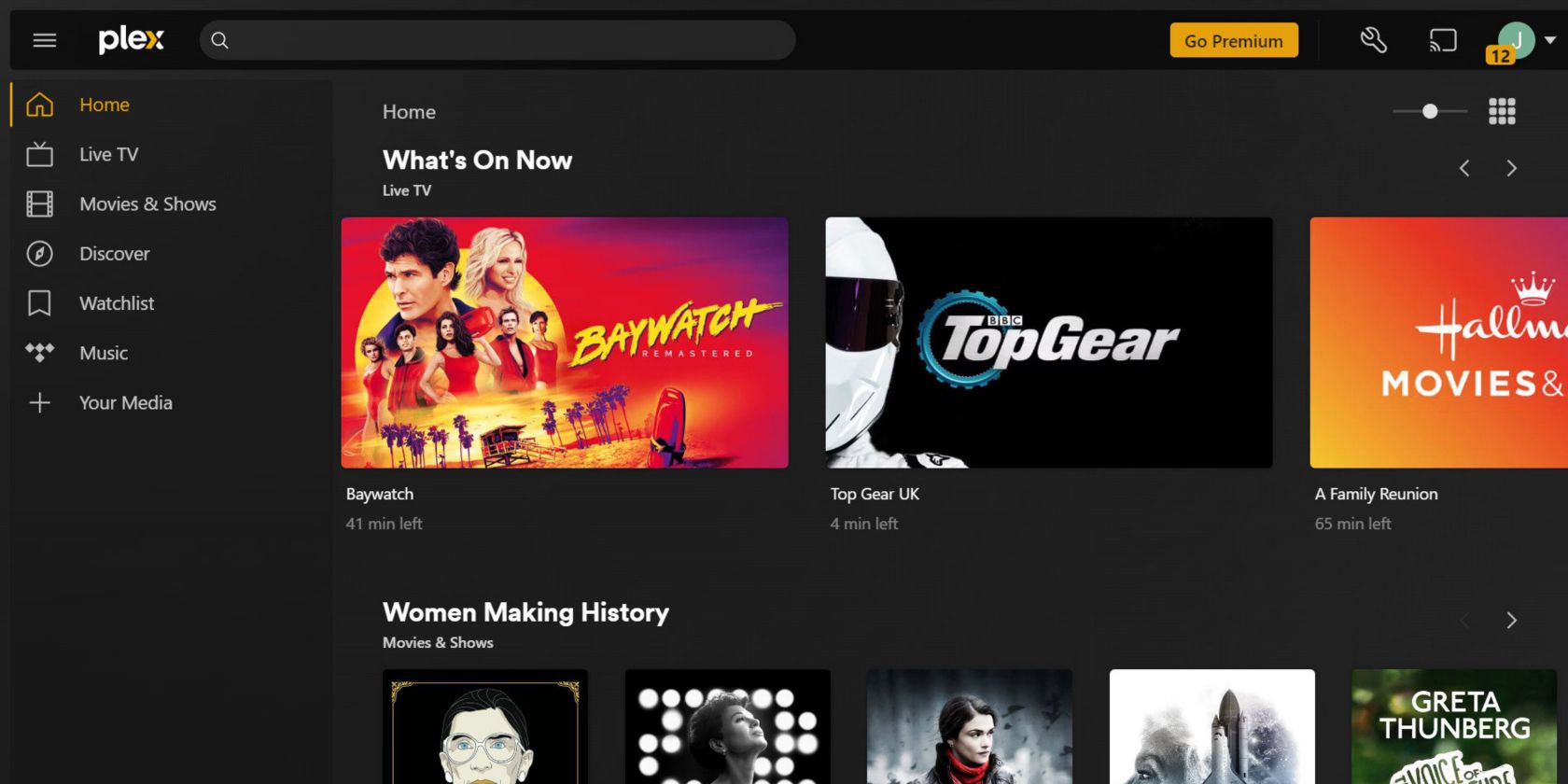This is a detailed screenshot of the Plex application interface, showcasing the "Go Premium" promotion. 

At the top, the screen features a black header with three horizontal lines indicating a menu, followed by the word "Plex." Adjacent to this, there is a search bar and, highlighted in gold letters, the phrase "Go Premium." Next to this, there appears to be an icon resembling a little screwdriver.

The main content shows the "What's On Now" section, which highlights currently available shows and movies. This includes "Baywatch," with 41 minutes remaining, "Top Gear," with 4 minutes left, and a Hallmark movie titled "A Family Reunion," with 65 minutes remaining. 

Underneath, there's a section labeled "Women Making History," featuring an image of Greta Thunberg and three other unidentified women. On the left side of the screen, the menu options are listed vertically, starting with "Home," followed by "Live TV," "Movies & Shows," "Discover," "Watch List," "Music," and "Your Media."

The user expresses unfamiliarity with the Plex platform.